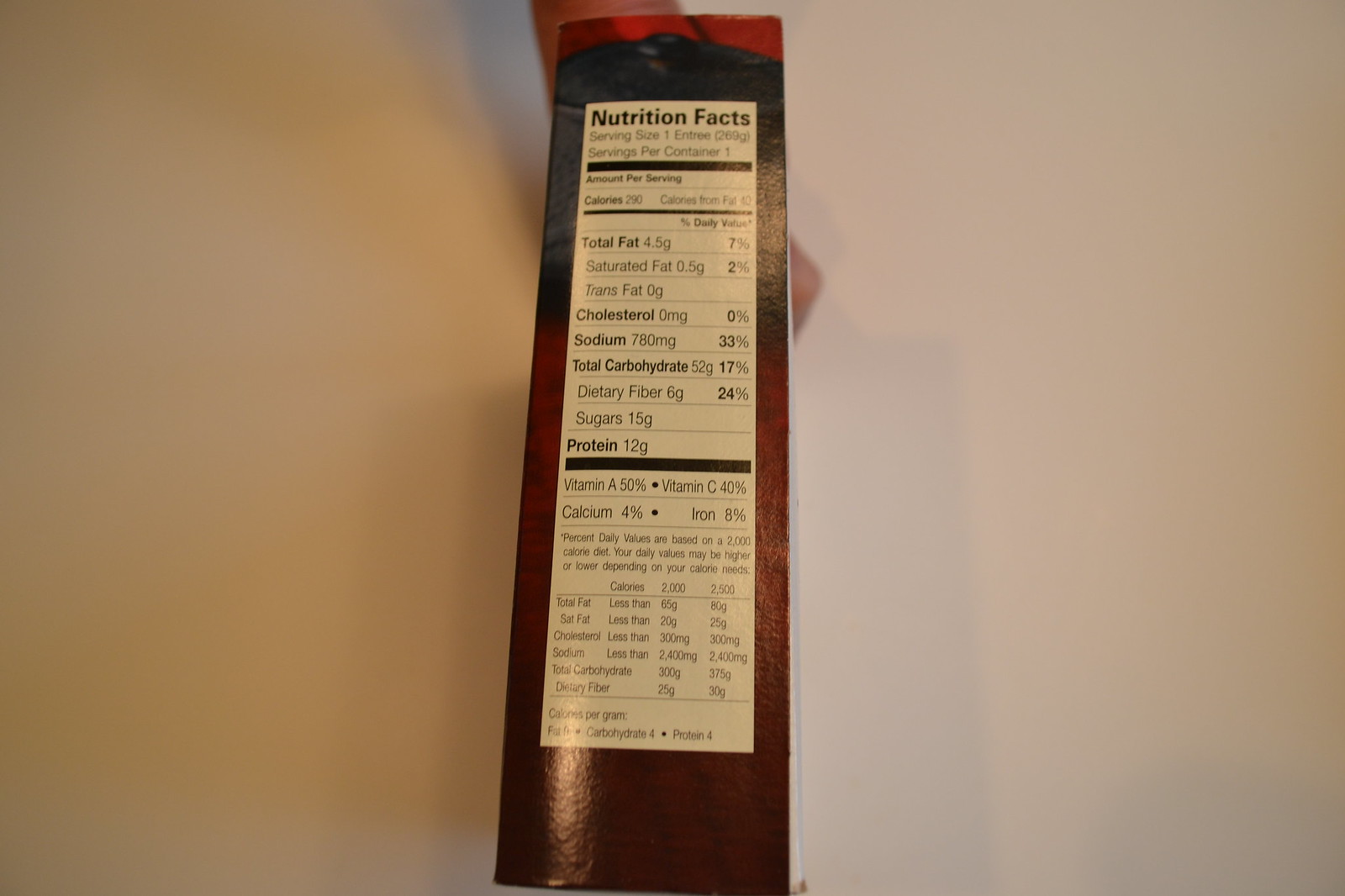This is an image of a nutritional facts label on the side of a brown box, set against a white wall in the background. The label itself is white and titled "Nutritional Facts" at the top. The details on the label include key dietary information:

- **Total Fat:** 4.5g
  - **Saturated Fat:** 0.5g
  - **Trans Fat:** 0g
- **Cholesterol:** 0mg
- **Sodium:** 780mg (noted as 7.8 in another line, likely an error)
- **Total Carbohydrates:** 52g
  - **Dietary Fiber:** 6g
  - **Sugars:** 15g
- **Protein:** 12g

The label also indicates significant percentages of daily values for various vitamins and minerals:
- **Vitamin A:** 50%
- **Vitamin C:** 40%
- **Calcium:** 4%
- **Iron:** 8%

At the very top, there's a section for serving size, but the text is too blurry to read. Below the nutritional details, there is some additional writing that is also too small and blurry to decipher.